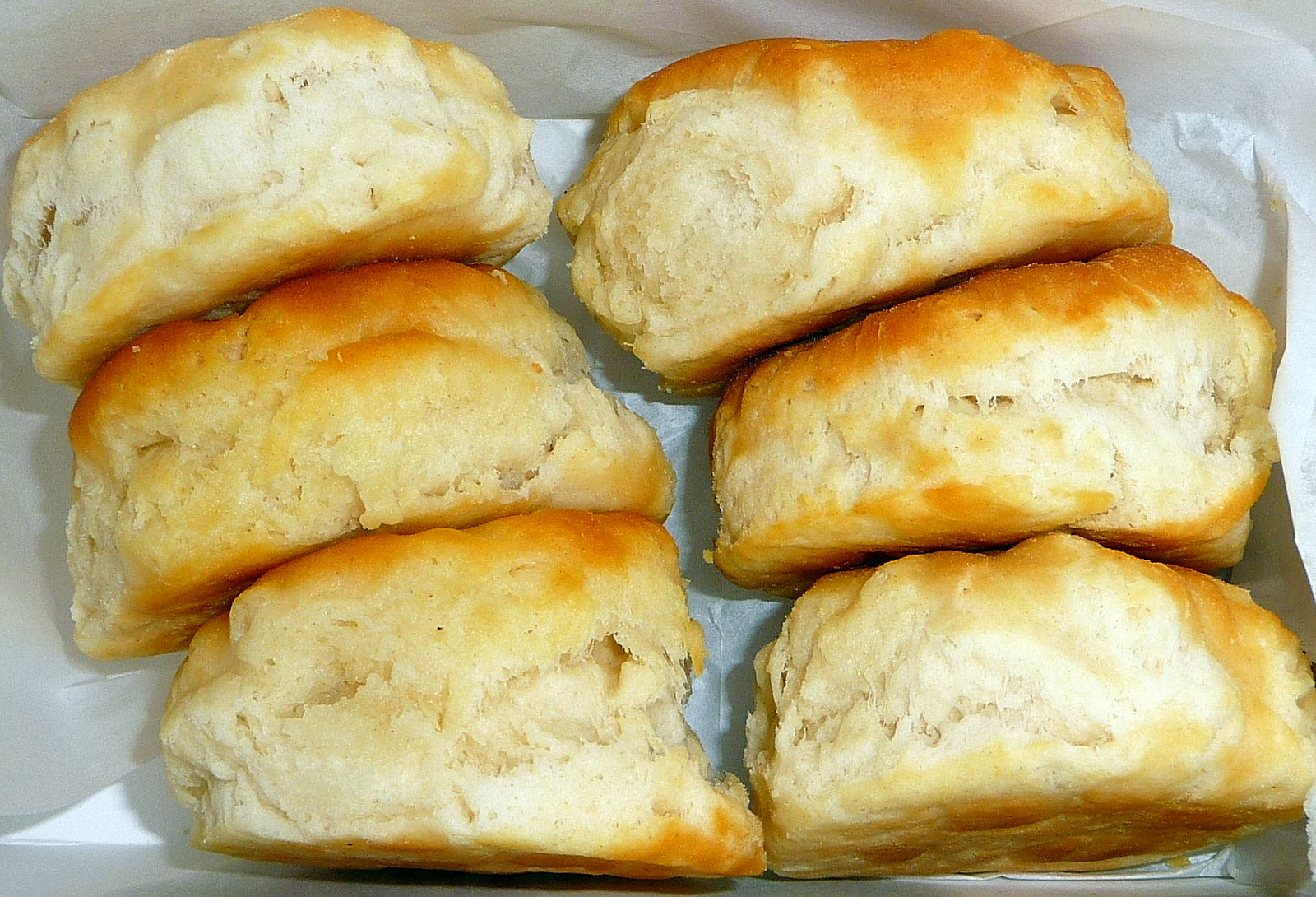This close-up colour photograph, in landscape orientation, features six delicious scones arranged in two vertical stacks of three each, nestled within white greaseproof paper. The golden-brown, crispy tops and bottoms of the scones contrast with their lighter, almost white, and yellow centers, indicating a perfect bake. The scones are positioned on their sides, revealing their flakiness and tempting texture. The packaging, which includes shiny cardboard edges on the front and right, suggests they were purchased from a bakery. The scones appear to be leaning slightly to the left within the container, enhancing the inviting, rustic appeal of this freshly baked treat.